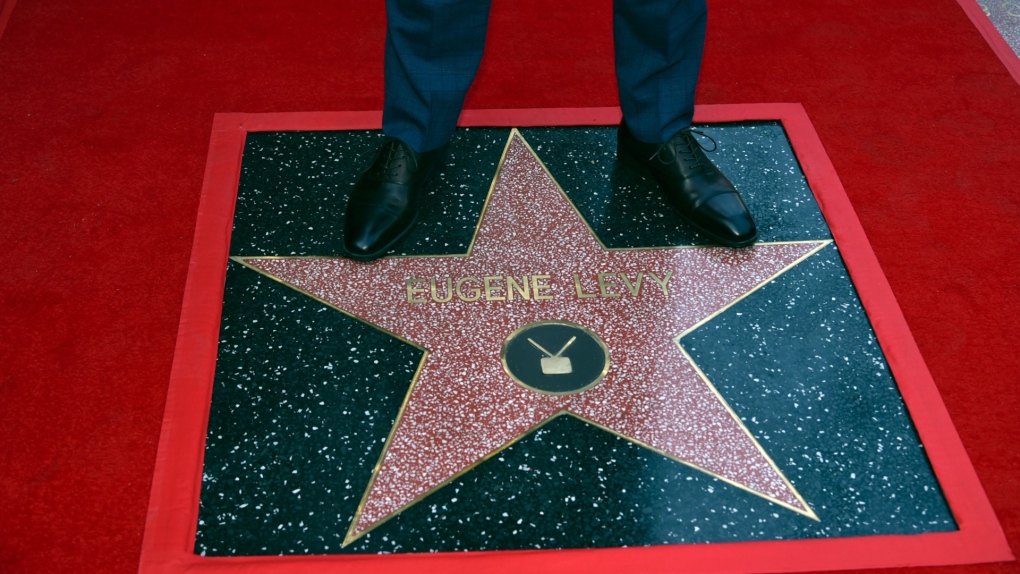In this detailed photograph, a person is dressed in polished black dress shoes and dark blue dress pants, standing prominently on Eugene Levy's star on the Hollywood Walk of Fame. The star, which celebrates notable figures in the entertainment industry, is set against a black, speckled background framed by a vibrant red outline, all laid over a luxurious red velvet carpet. The star itself is a striking red speckled with white and bears Eugene Levy's name in gold. Beneath his name is a golden circular medallion featuring a stylized television with antennae. This medallion signifies Eugene Levy's contributions to the television industry. Each foot of the person in the photograph rests elegantly on opposite sides of the star, highlighting the momentous occasion of the star unveiling.